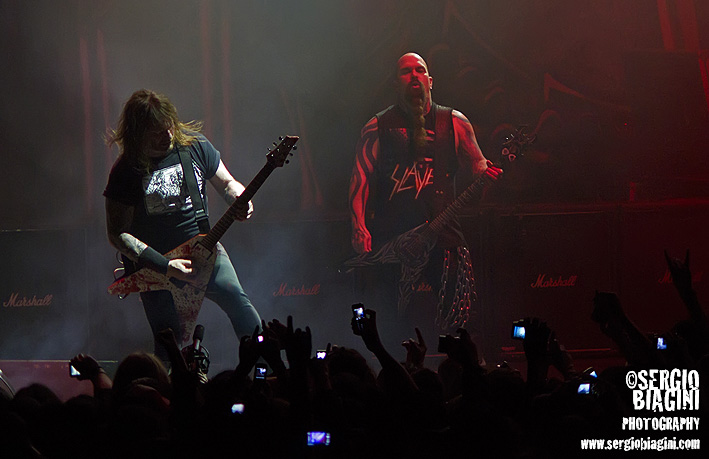This is a color photograph of a live rock concert featuring the legendary band Slayer, captured indoors. In the foreground, the band's guitarists are prominently displayed. On the left, the guitarist with long brown hair cascading past his shoulders is dressed in a black graphic t-shirt and blue jeans. On the right stands Kerry King, recognizable by his bald head, extensive arm tattoos, and the chains dangling from his belt. King is illuminated by a white spotlight while playing a white electric guitar splattered with fake blood. The other guitarist, bathed in a red spotlight, is equipped with a grayish guitar. Behind them, a towering stack of Marshall Amps emphasizes the raw power of the performance. The audience is fully engaged, with many attendees recording the electrifying event on their phones. Across the bottom of the image, the text “Sergio Bianchini Photography, www.sergiobianchini.com” credits the photographer. The shared communal energy of capturing the concert on phones indicates a moment that is both personal and collective for the fans.